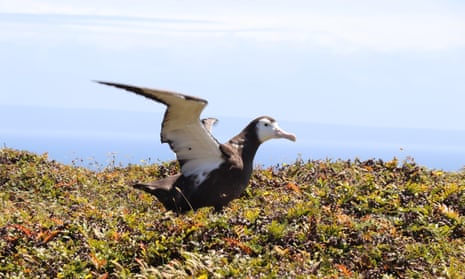In this detailed image, we see a bird, possibly a duck, with its wings fully extended upwards as if preparing to take flight. Its plumage is predominantly black, with contrasting white feathers visible underneath its wings and a white face. The bird has a distinct white beak and piercing black eyes. It is perched on a grassy area, suggesting it is stationed on solid ground. The background reveals an overcast sky with some clouds, indicating a potentially hazy day but with sunlight present, as evidenced by the shadows and reflections seen on the bird. Spanning behind the bird is a vast expanse of water, likely the ocean, adding to the scene's serene, open atmosphere. The location appears to be near a beach or coastline, with a faint, possibly mountainous or hilly landmass in the distance. This comprehensive view of the bird captures about 40% of the image in focus, amidst a somewhat pixelated and low-resolution photograph.